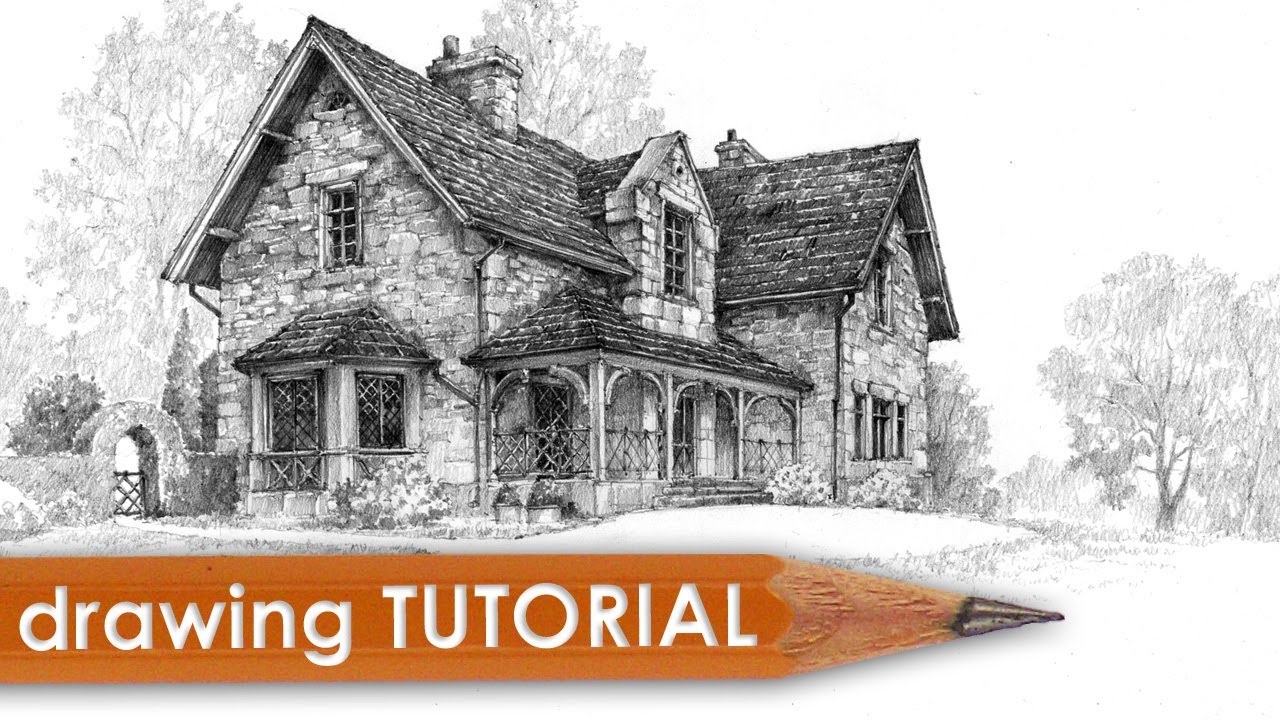The image is a color photo featuring a detailed black and white pencil sketch of an old stone or brick cottage with a shingled roof and multiple architectural elements. The cottage, centered in the image, has an arched gated entryway, a bay window, a smaller window above it, and two chimneys. Surrounding the house are light-shaded pencil-drawn trees, a manicured hedge, and small flowers. In the foreground, a large yellow pencil with a sharp point is superimposed at the bottom, bearing the text "drawing tutorial" in white lettering, with "drawing" in lowercase and "TUTORIAL" in uppercase. The entire scene resembles an English countryside setting with intricate details like crosshatched windows and a picturesque porch with archways, all rendered in a purely monochromatic palette with varying shades of black and gray.